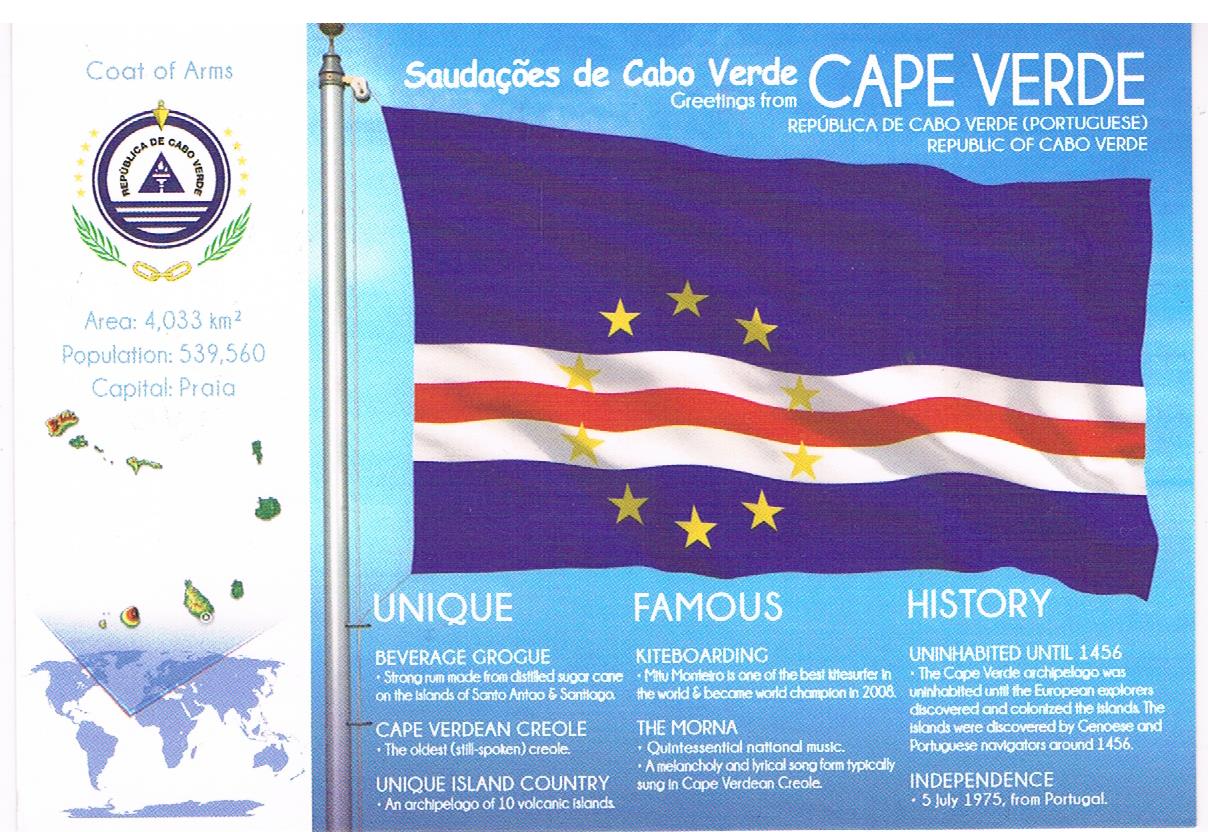The vibrant poster for Cape Verde features an informative mix of imagery and text highlighting the unique attributes of the island nation. Along the left edge, a vertical white bar runs the full height, displaying the coat of arms of the Republic of Cabo Verde prominently at the top. Below it, detailed statistics include the area of 4,033 square kilometers, a population of 539,560, and the capital city, Praia. 

A map showcases the 10 volcanic islands of the archipelago, pinpointing Cape Verde's location in the world. The flag, predominantly blue with a white-red-white ribbon at the bottom and a circle of stars reminiscent of the European Union, occupies the right side of the graphic. The top portion of the poster contains text in both Portuguese and English, stating "Sadaqus de Cabo Verde," "Greetings from Cape Verde," and "Republica de Cabo Verde."

Further, the poster features sections highlighting the country's unique aspects, famous elements, and historical milestones. Under "unique," it describes Cape Verde's renowned beverage, strong rum made from distilled sugarcane on Santo Antão and Santiago islands, as well as the Cape Verdean Creole, the oldest still-spoken Creole language. The "famous" section celebrates the country's kiteboarding culture, noting Mitum Monteterreiro, a world champion kite surfer in 2008, and the Morna music, a melancholic and lyrical song form sung in Cape Verdean Creole. The "history" section notes that the archipelago was uninhabited until discovered by European explorers around 1456 and gained independence from Portugal on July 5, 1975. The combination of these elements paints a vivid picture of Cape Verde’s rich culture, history, and natural beauty.